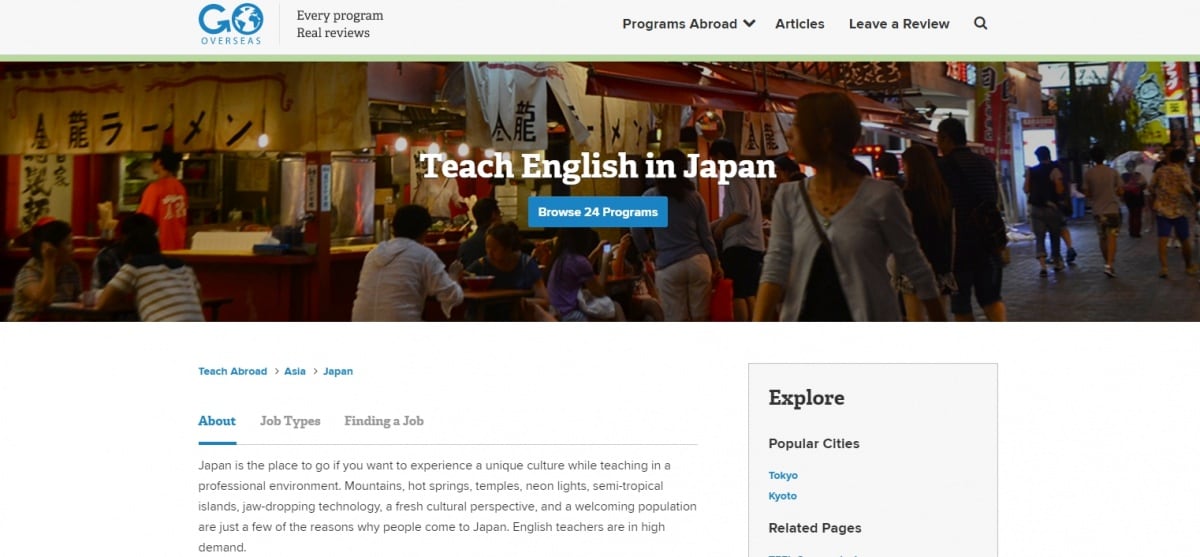This screenshot captures a section of the website "Go Overseas." It showcases an array of features, including program reviews for overseas ventures and a prominent search bar. The main focus is on a segment titled "Teach English in Japan," which highlights 24 available programs. 

The accompanying picture introduces a vibrant scene set in an Asian market. Predominantly filled with people of Asian descent, the image portrays individuals leisurely exploring the market. Some patrons are seated at tables, enjoying their meals and beverages, while others meander through the bustling pathway. The market is nestled within a spacious hall, characterized by its high ceilings and lined with various shops along the corridor, culminating in a visible doorway at the far end.